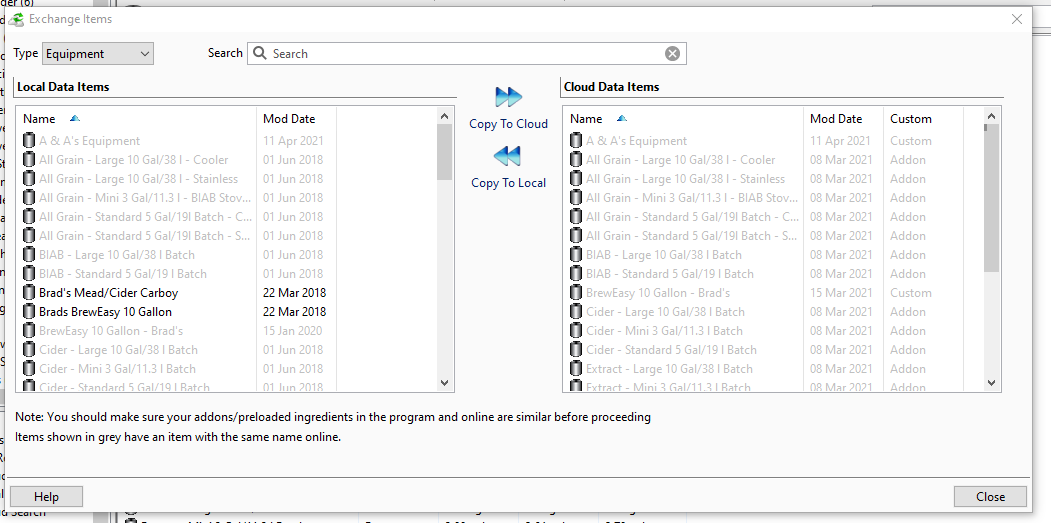**Detailed Caption:**

Displayed is an administrative panel titled "Exchange Items," appearing as a modal overlay. The title "Exchange Items" is prominently positioned in the upper left corner of the panel. Below the title, there is a section labeled "Type Equipment," accompanied by a search option for user convenience.

The panel is divided into two primary columns. The left column is titled "Local Data Items," and the right column is titled "Cloud Data Items." Between these columns are two sets of directional arrows. The first set, with arrows pointing to the right, is labeled "Copy to Cloud," while the second set, with arrows pointing to the left, is labeled "Copy to Local." These arrows facilitate the transfer of items between local and cloud databases.

Each column lists items with the headers "Name" and "Mod Date" (Modification Date). In the "Local Data Items" column, an entry labeled "ANA's equipment" is dated April 11th, 2021. Correspondingly, in the "Cloud Data Items" column, there is a similar entry, but with an additional label, "Custom," following the date. Both entries appear grayed out, indicating a special status or condition.

Further down the "Local Data Items" column, highlighted entries include "Brad's Meats Cider Carb Glory" and "Brad's BrewEasy 10-Gallon," both dated March 22nd, 2018. Notably, these items do not have equivalent entries in the "Cloud Data Items" column, and their appearance is also gray, suggesting a specific context or status.

At the bottom of the panel, a note advises users to ensure that their add-ons, pre-loaded ingredients, and programs are consistent online and offline before proceeding. An explanation clarifies that gray indicates items with identical names online.

Below this note, a thin black pixel line demarcates the informational section, followed by two buttons at the panel's bottom corners: a "Help" button on the lower left and a "Close" button on the lower right, both in gray.

This detailed description encapsulates the functionalities and visual elements of the Exchange Items administrative panel, highlighting the interactive elements and the contextual guidance provided to the user.